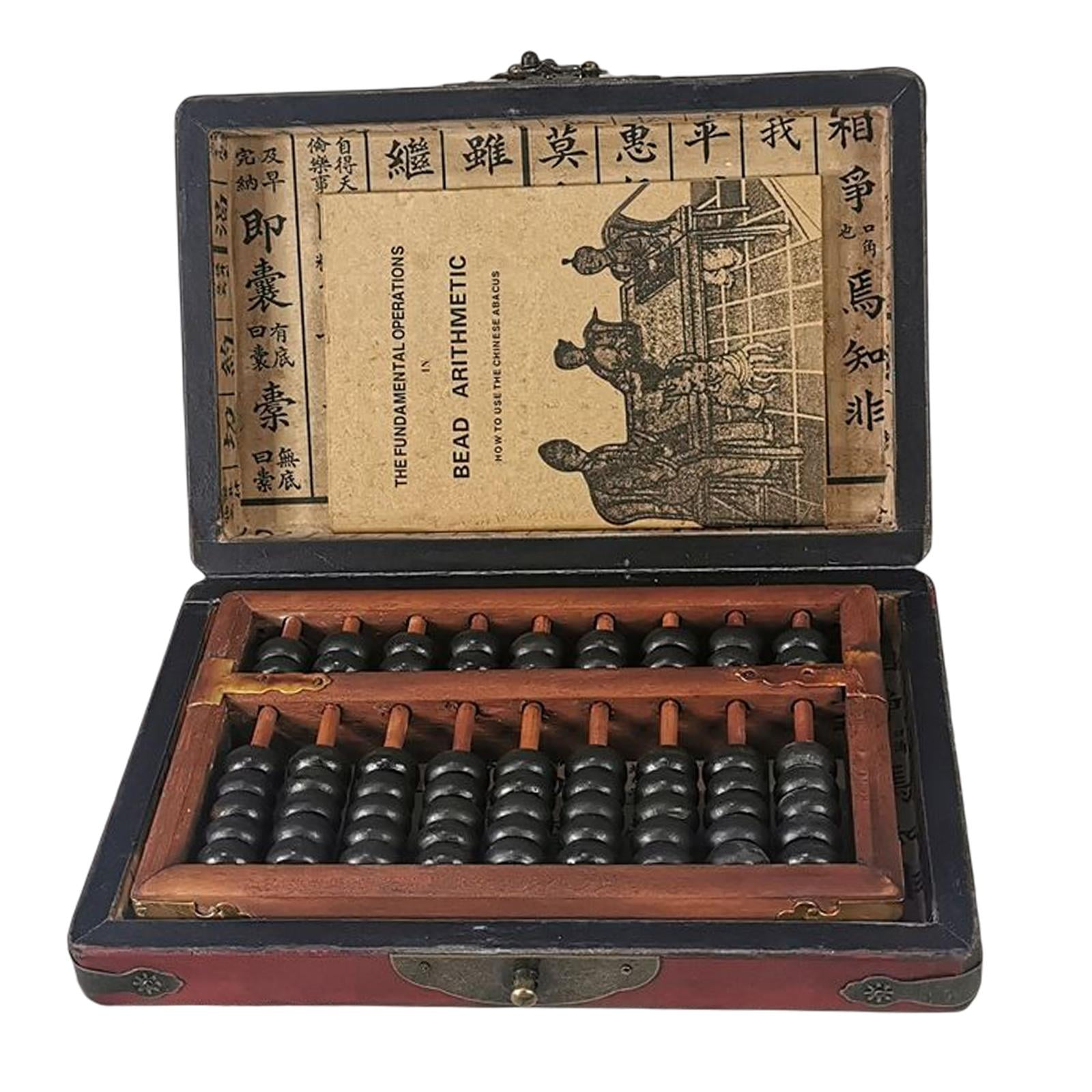This is a detailed photograph of a vintage Chinese abacus set against a stark white background. The abacus, a traditional bead counting calculator, is encased in a red-painted wooden carrying box with metal clasps and hinges for secure closure. The abacus, which can be removed from the box, features two rows with nine columns: the top row contains two black beads per column while the bottom row contains five black beads per column. When the box is opened, a multi-lingual booklet titled "Fundamental Operations in Bead Arithmetic" is revealed, providing instructions on how to use the abacus. The booklet also contains an illustration depicting a Chinese man, woman, and boy seated around a table, engaging in the use of the abacus. The meticulous design and vintage appearance of the set suggest it was intended for educational purposes to teach arithmetic.